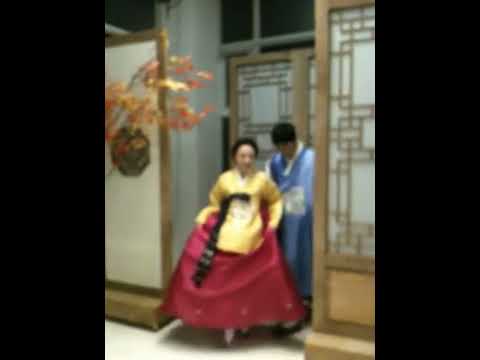In this photograph, a young Asian couple is prominently featured, moving through an ornate doorway that suggests traditional Asian influence. The woman is positioned at the center, stepping forward in a vibrant ensemble consisting of a wide, bright red skirt and a long-sleeved yellow top accented with a black sash around her waist. Her dark hair is partially pulled back from her face, and she holds up her red skirt slightly. To her left, just behind her shoulder, the man is seen in a light blue formal suit with white details, including a white shirt underneath. His head is slightly bowed as he appears to be escorting the woman, possibly down a step or out of a doorway.

The background features heavily decorated wooden screens with glass or decorative panels forming squares and rectangles. On the left side of the image, there is a vine-like plant growing from a wall sconce, partially overhanging the couple. A small branched tree with orange fruit is visible next to the doorway, enhancing the traditional aesthetic. The scene captures a moment that is both festive and formal, with the couple possibly dressed in regional attire. Given the detailed background and ornate surroundings, the setting evokes an air of cultural richness, suggesting an indoor or transitional indoor-outdoor space.